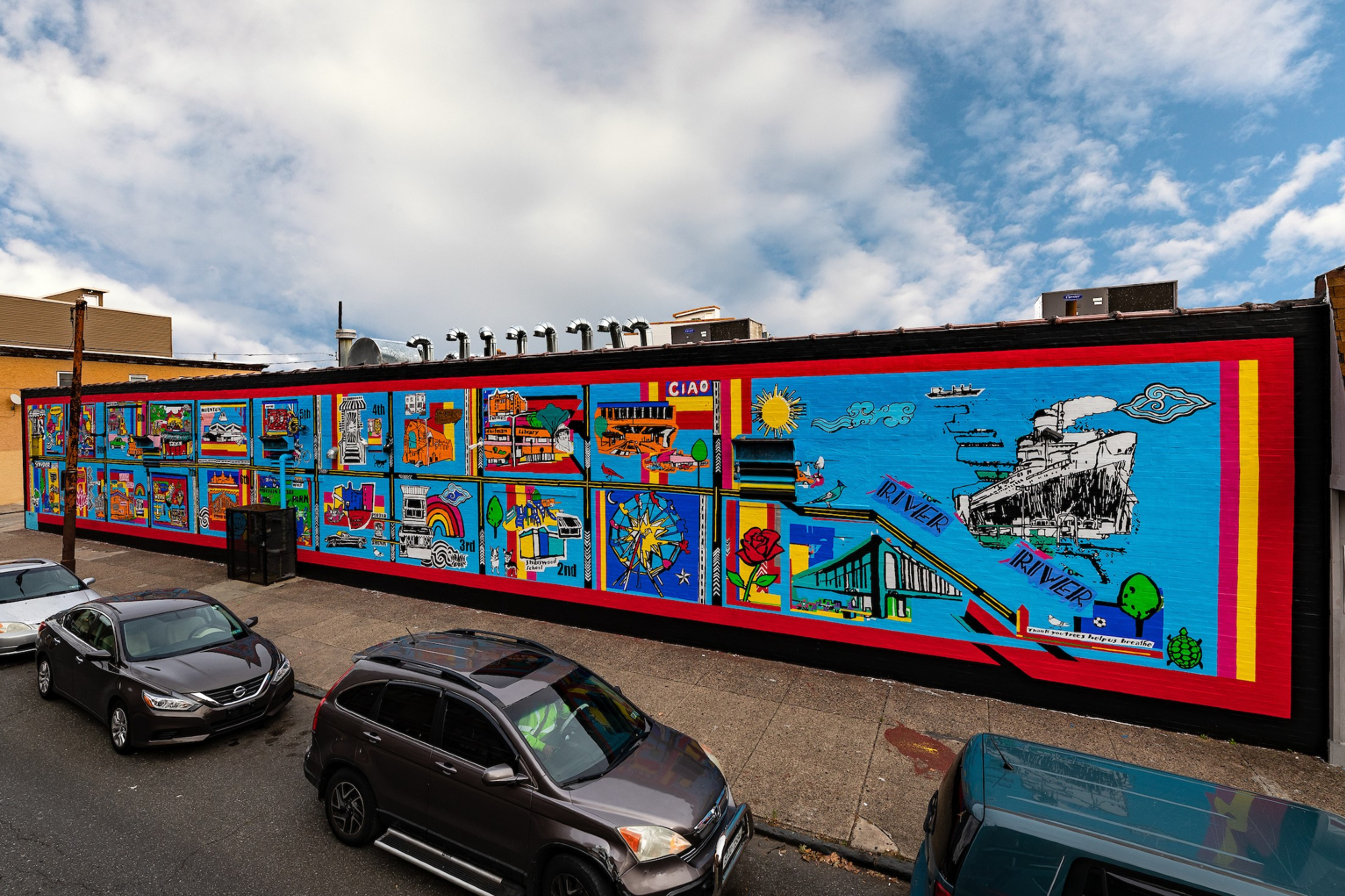This photograph captures a wet city street lined with parked cars next to a concrete sidewalk. The focal point is a long, rectangular building with a striking mural covering its brick wall. The mural, framed by a red border, features numerous panels primarily in blue, depicting various scenes connected by a river theme. 

The mural includes illustrations of a steam liner labeled "river" in a blue backdrop, a yellow sun, and a green suspension bridge. Interspersed among these are images like a cruise ship, a turtle, a tree with a red rose, and a rainbow. The sky above the mural is painted blue with white clouds.

Details of distant mural panels are blurry, but the diversity of scenes adds vibrant color to the industrial building with its flat roof and silver exhaust pipes. Additional street features include a rusty street light, a black trash can, and a yellowish building with a brown roof in the background, partially cut off. The photograph vividly captures the essence of the moment, emphasizing the colorful artwork juxtaposed against the dull, rainy street.